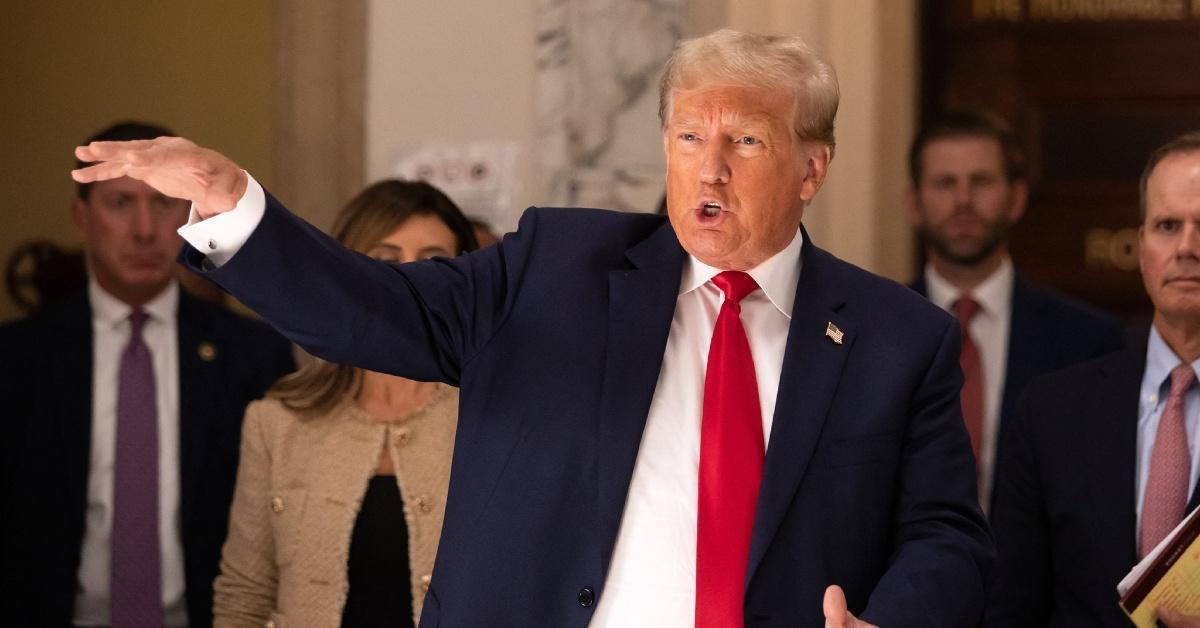In this indoor image set in what appears to be an important political building with beige walls, former President Donald J. Trump, distinguished by his orange-tinted skin, stands as the focal point. Attired in a blue suit jacket adorned with an American flag pin, a white collared shirt, and a red tie, Trump is speaking, likely addressing the press. His lips are parted as if mid-sentence while one hand is raised in a gesture. Surrounding him are individuals dressed in formal business attire, including white shirts, ties, and suit jackets, along with women in business casual clothing, contributing to the formal and significant atmosphere of the scene. This moment captures Trump passionately advocating for the rights of American citizens and emphasizing his efforts to avoid international conflicts during his tenure, contrasting with the increased number of wars and loss of freedoms around the globe that some attribute to his absence from office.